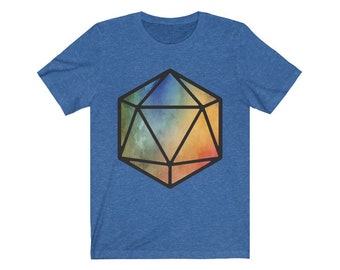The image depicts a medium blue short-sleeved T-shirt with a round neckline, featuring a prominent central design of a multi-faceted 3D shape that heavily resembles a 20-sided die, commonly associated with Dungeons & Dragons. The geometrically complex figure, constructed from triangles, is vividly colored with a spectrum ranging from dark blues and greens to yellows, reds, and oranges, giving it an impression of light reflection. The intricate design covers a significant portion of the shirt's front, adding a vibrant and eye-catching contrast against the plain cotton fabric of the T-shirt. The depiction appears highly detailed, almost like a 3D model with black lines outlining the polygons that compose the structure.